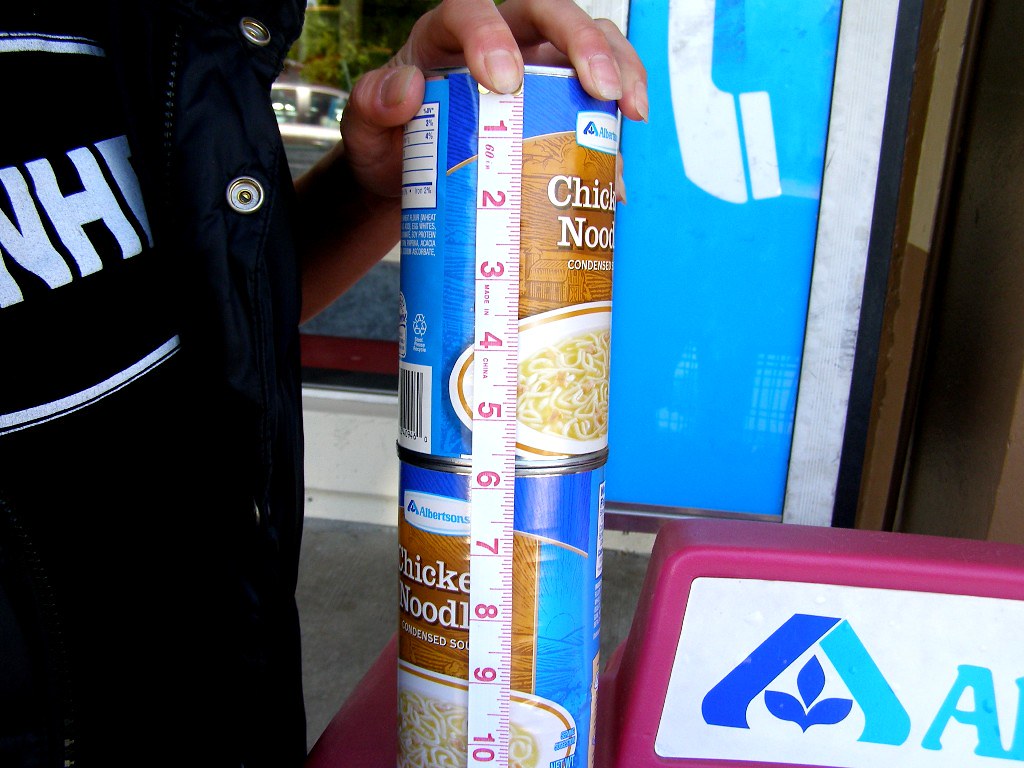A man measures the height of a stack of two Albertson's condensed chicken noodle soup cans using a white tape measure. The man is partially visible, wearing a black T-shirt with white block lettering and an oval design, covered by a black jacket equipped with a zipper and snap closures for wind protection. His left hand steadies the cans, which feature a blue label with a brown section displaying a picture of a bowl of chicken noodle soup—white with a gold rim.

The tape measure indicates the stack stands approximately 10.5 to 11 inches high, though the measurement isn't entirely clear as the tape is clipped near the bottom. Behind the cans, there is a pole-mounted payphone in a white privacy enclosure with a blue rectangle and phone handset icon. Additionally, a purple sign displaying part of the Albertson's logo ("AL...") is visible, matching the branding on the soup cans. The purpose of the measurement remains unclear.